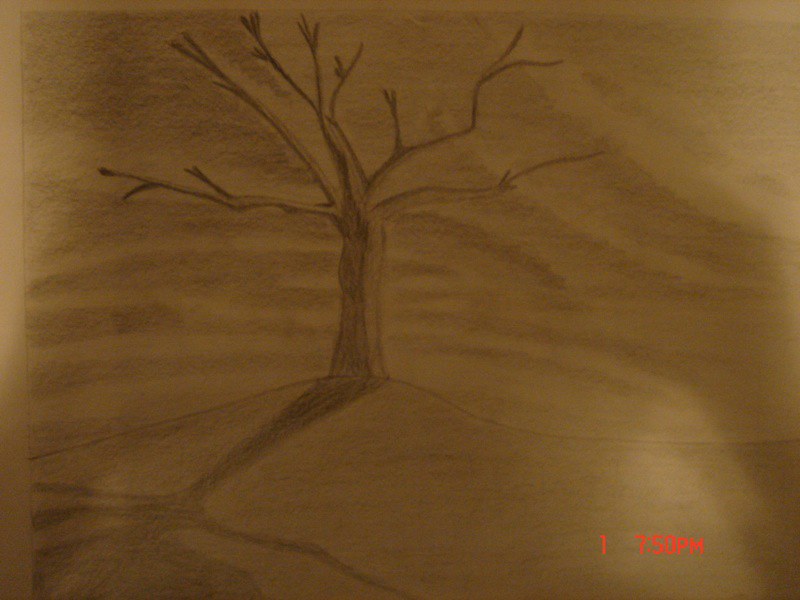The image is a dimly lit photo of a pencil sketch on white paper, giving it a sepia-toned appearance. The sketch depicts a large, leafless tree with five prominent branches—three extending to the left and two to the right. The tree stands on a slight hill that curves upward toward the tree before descending to the right. The background is shaded in pencil, revealing visible pencil lines and hints of faded clouds. A shadow from the tree falls toward the bottom left, enhancing the depth of the scene. In the bottom right corner, there is a red digital time stamp reading 7:50 p.m., adding a modern touch to the otherwise rustic artwork.